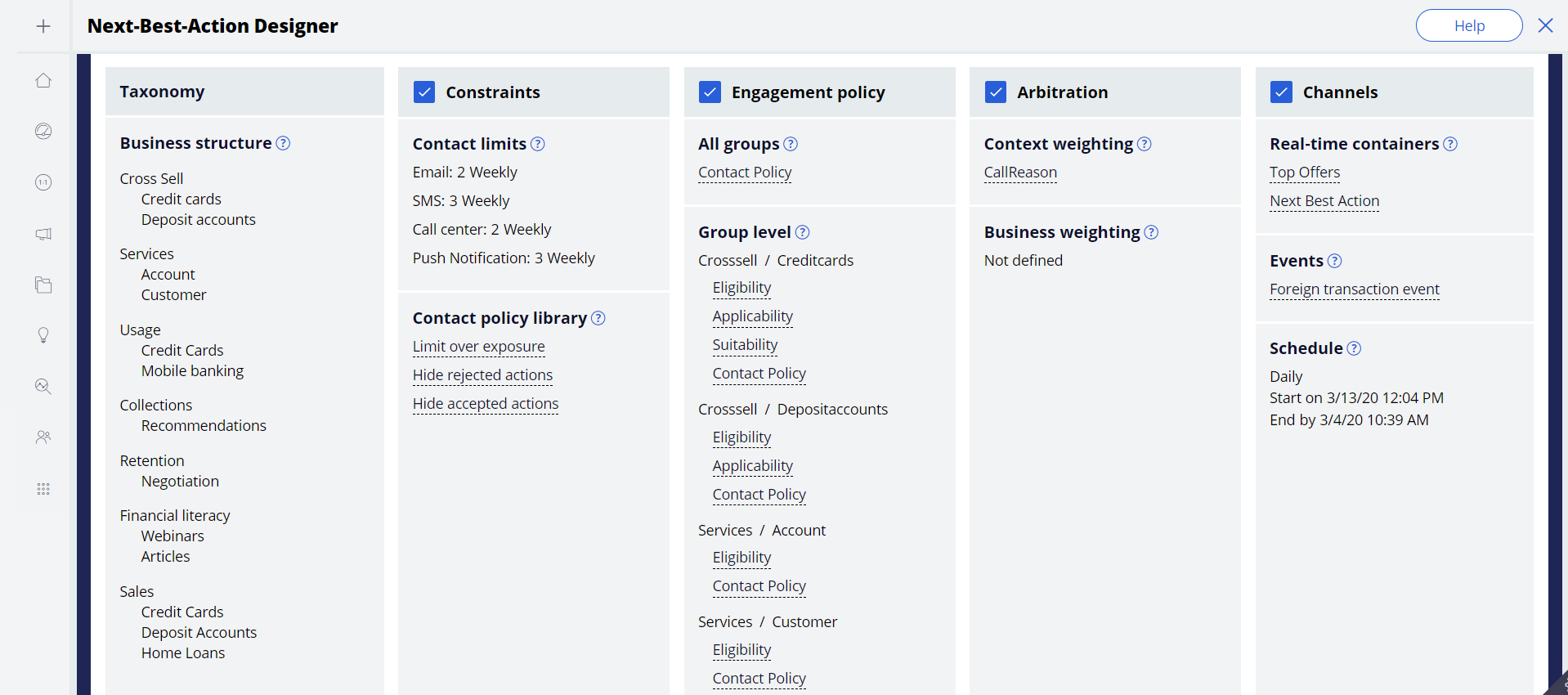This image is a detailed screenshot of the "Next Best Action Designer" interface, seemingly taken from a webpage. On the right side of the screen, there is a navigation bar featuring several icons and options. At the top of the navigation bar, there is a home icon and a magnifying glass icon for search functionality. Below these icons, the navigation options are listed, each accompanied by a blue checkbox.

The listed options are as follows:
- **Taxonomy**
- **Business Structure**

Following these sections, under the **Constraints** heading, the specific contact limits are detailed:
- **Email:** Limited to two contacts per week
- **SMS:** Limited to three contacts per week
- **Call Center:** Limited to two contacts per week
- **Push Notification:** Limited to three contacts per week

Additionally, the Constraints section includes:
- **Contact Policy Library**
- **Limit Overexposure**
- **Hide Rejection**
- **Hide Accept Actions**

Under the **Engagement Policy** section, the terms are:
- **Contact Policy**
- **Group Level**
- **Eligibility**
- **Suitability**
- **Contact Policy for Cross Sale**
- **Eligibility**
- **Applicability**

In the **Arbitration** category, the interface lists:
- **Context Weighting**
- **Business Weighting**

Finally, the **Channels** section includes:
- **Real-Time Containers**
- **Events**
- **Schedule**

The interface appears to be designed for detailed and structured management of engagement policies, contact constraints, and arbitration processes within a business context.